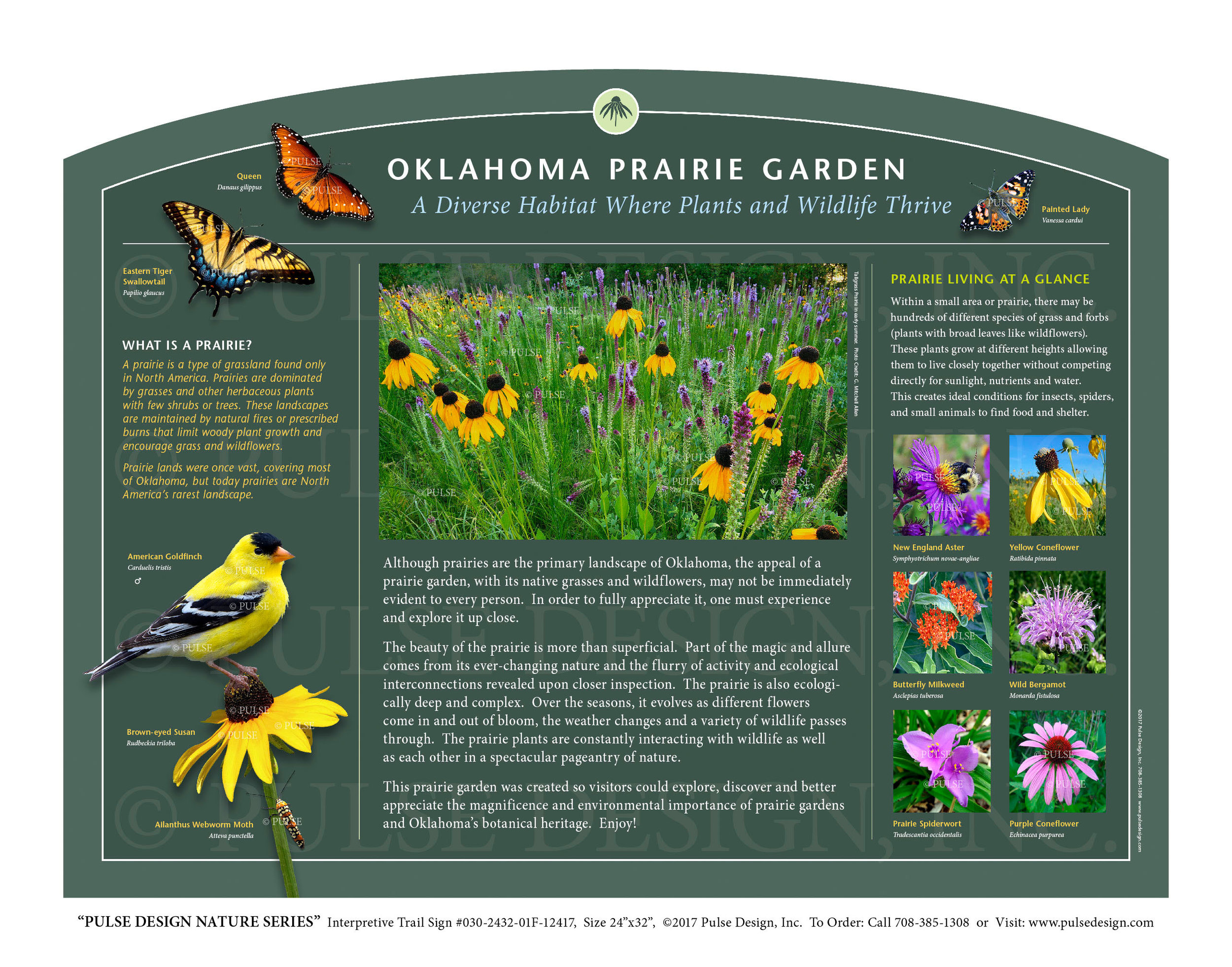The image is a detailed poster titled "Oklahoma Prairie Garden" at the top in white text, followed by the subheadline "A diverse habitat where plants and wildlife thrive." The poster is mainly green with a rectangular shape, curving upward at the top side. It is divided into three sections, with illustrations and photographs of various elements of the prairie ecosystem.

The left side of the poster features an orange and yellow butterfly with the text "What is a prairie?" in white, followed by the definition in yellow text: "A prairie is a type of grassland found only in North America. Prairies are dominated by grasses and other herbaceous plants, with few shrubs or trees."

The central section showcases vibrant paintings and photographs of wildlife. Particularly, there are colorful depictions of butterflies—one bright orange and yellow, another yellow with blue. Below these, there is a photograph of wildflowers resembling black-eyed Susans, surrounded by what appears to be a field of lavender.

To the right is a column titled "Prairie Living at a Glance," which describes various flowers in the garden through six pictures with accompanying descriptions. Additionally, this section includes an illustration of a goldfinch perched on a flower bulb, with an insect climbing up the stalk, though the lettering beside the image is small and partially unreadable.

At the bottom of the poster, small text reads "Pulp's Design Nature Series," along with detailed dimensions of the poster. The overall design intricately describes the prairie ecosystem, making it an engaging and informative piece.